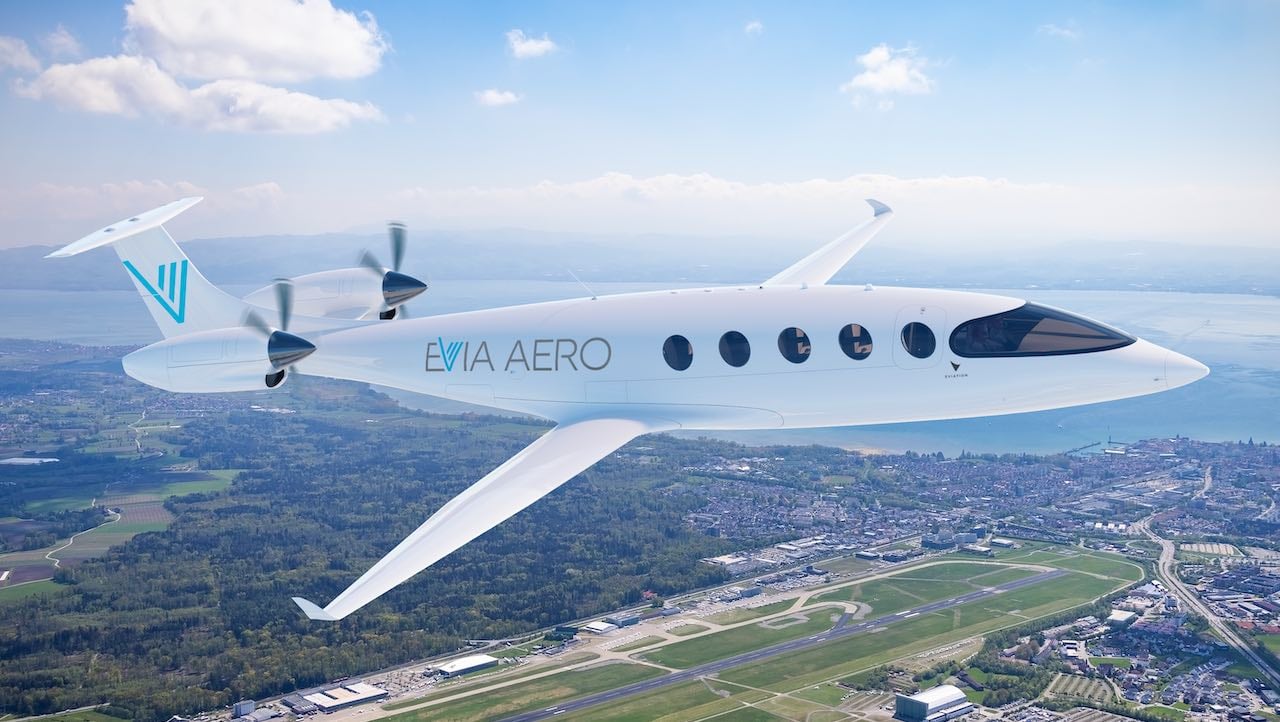A sleek, white airplane with the name "EVIAERO" emblazoned on its side, featuring a distinctive blue 'V' on the tail, soars high above a picturesque landscape. This unusual aircraft, notable for its propellers positioned at the tail, cuts through the clear, bright sky dotted with a few hazy clouds. Below, a rich tapestry of scenery unfolds: expanses of green grass and trees, a small airport with a visible runway, and a quaint village bisected by a major road. Further in the distance, a body of water – possibly a river or ocean – can be seen, separating two land masses under the brilliant sunshine. The airplane itself stands out with its narrow wings, pointed nose, and twin fans at the tail, a unique design suggesting a modern, possibly electric-powered flight.